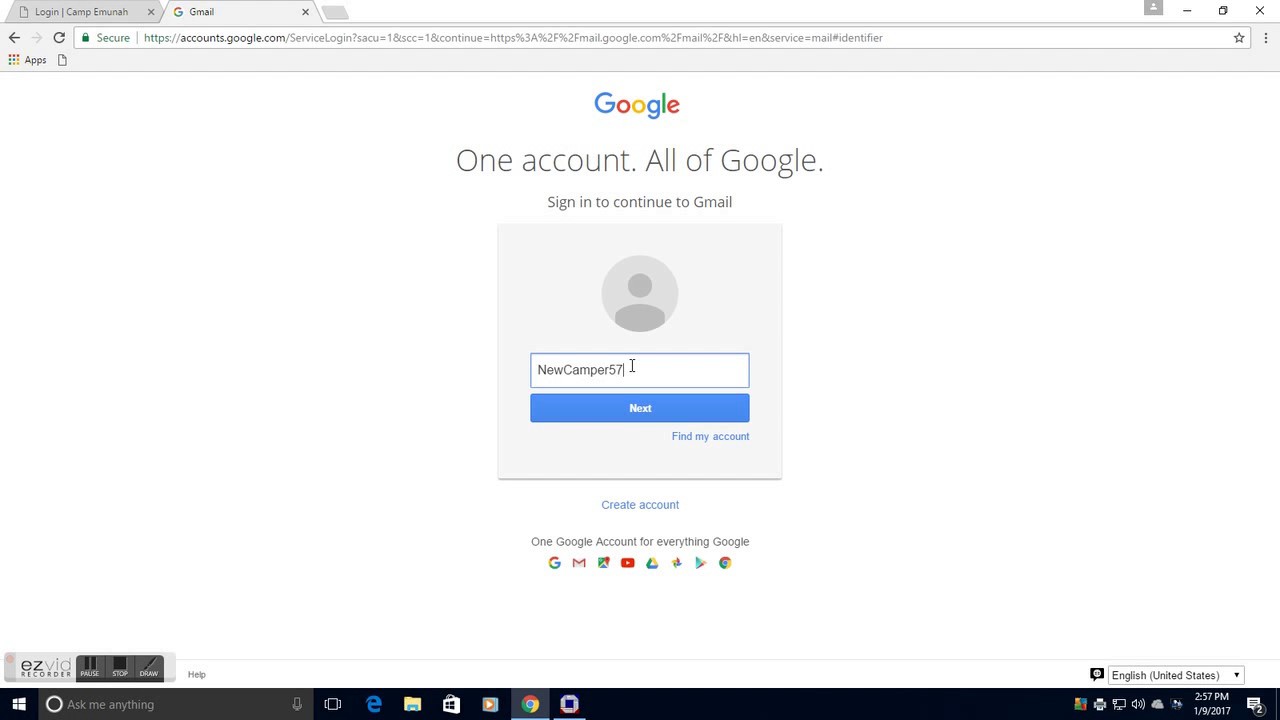This screenshot captures the desktop of a Windows computer, identified by the black toolbar at the bottom of the screen featuring the Windows logo on the far left. The toolbar includes various pinned icons and offers a search or assistant query option. On the right side of the toolbar, the current time and various notifications are displayed.

The primary focus of the screenshot is an open Google Chrome browser window. The user has two tabs open; the active tab is Gmail, while the other tab is titled "Login for Camp Yuma." The background of the Chrome window is predominantly white with hints of light gray. 

On the Gmail tab, the topmost element is the multicolored Google logo. Below this, in black font, it reads "One account. All of Google." Following this is the prompt "Sign in to continue to Gmail." Below the prompt is a light gray circle with an avatar, indicating a user login session. Underneath this, a white input box for the username or email address shows the partially entered text "New Camper 57." Beneath the input box, a blue "Next" button awaits further interaction.